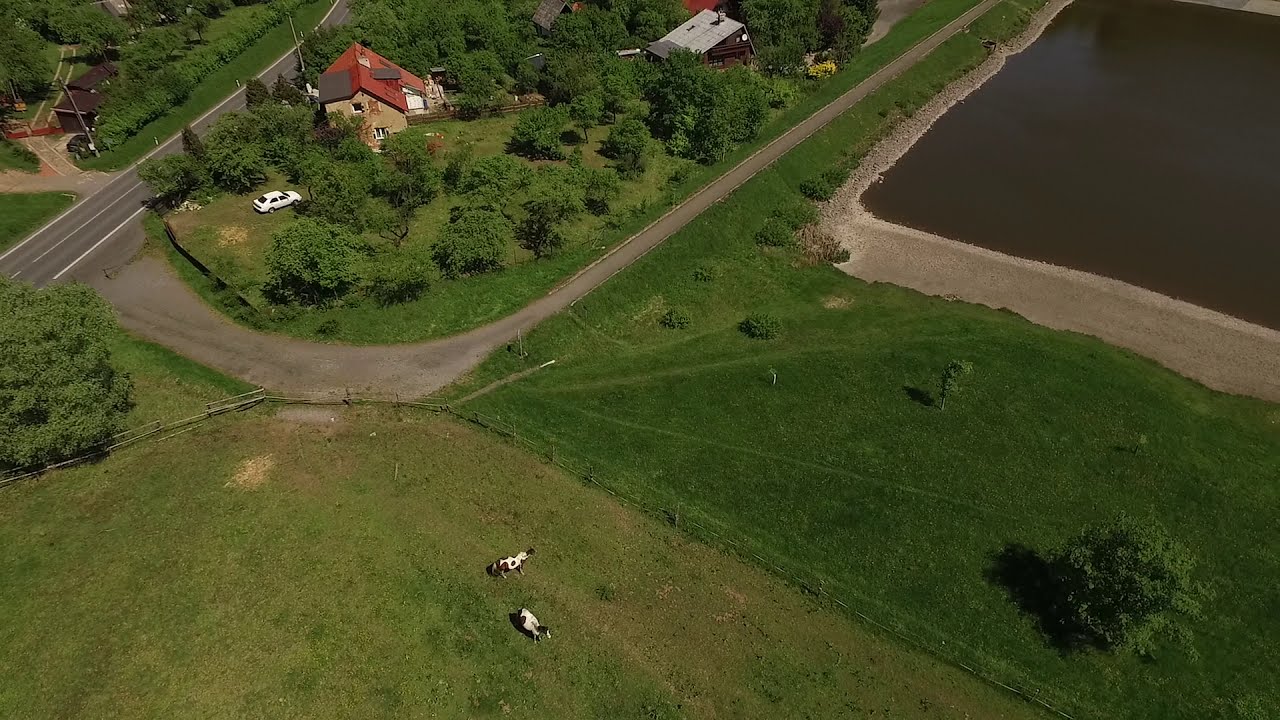This top-down daytime image captures a rural setting featuring a variety of elements. At the top of the image is a brown building with a triangular red roof, complemented by green trees and a white car parked in front. Adjacent to this house is another with beige walls and an orange roof, possibly equipped with solar panels. On the left and right sides of the houses, roads traverse the landscape.

In the lower section of the image, a fenced-in grassy field is home to two white and brown spotted cows standing close to each other. Adjacent to this area, on the right, is a grassy field intersected by a brown, muddy square corner of a lake surrounded by dark brown sand dunes. There are two black and white clouds near the bottom, adding a touch of contrast to the gray grassland. In the top right corner of the image, a square area of brown land is visible, contributing to the rustic atmosphere. Overall, the serene environment is meticulously maintained, from the mowed grass to the carefully placed elements.